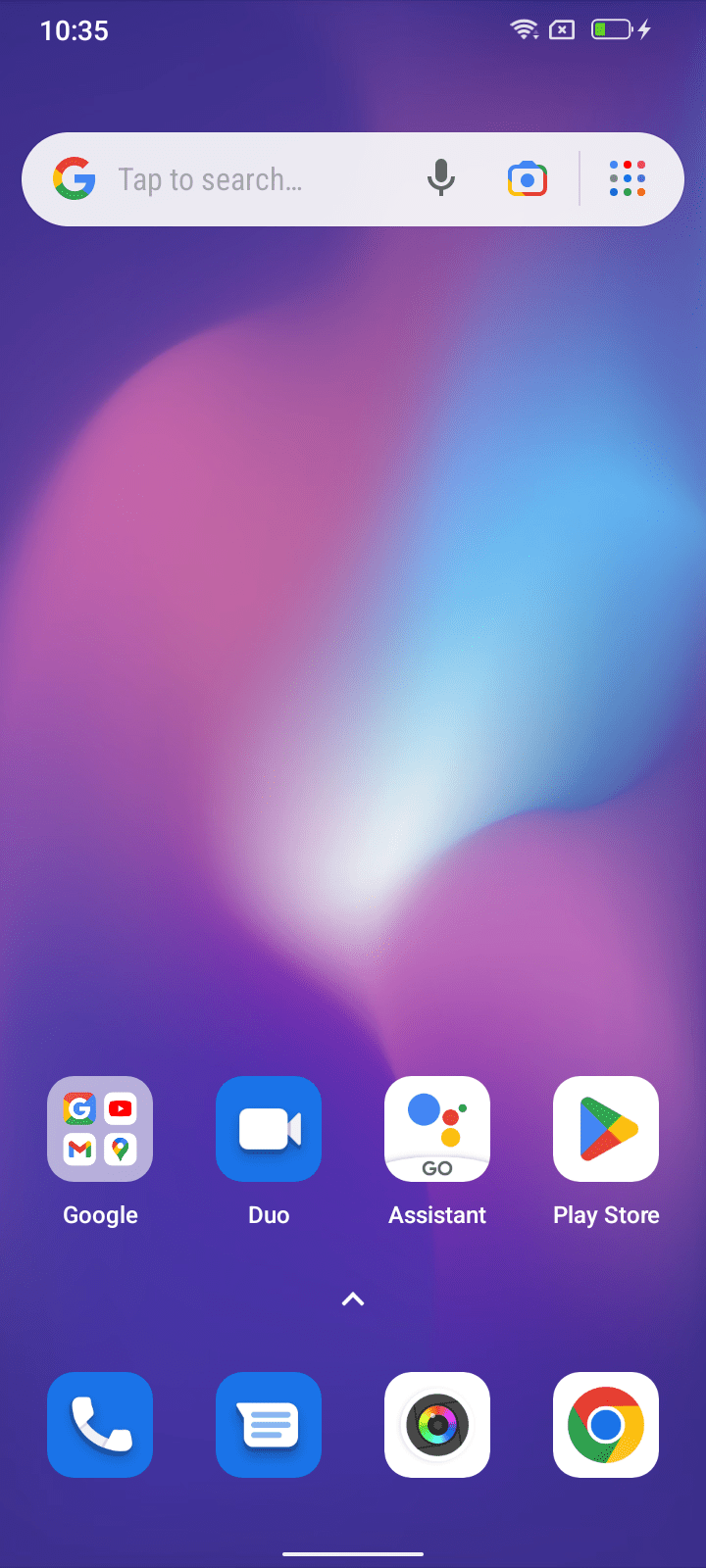This screenshot appears to have been captured from an Android smartphone. At the very top of the screen, the status bar shows the time as 10:35 alongside a Wi-Fi icon and a battery icon displaying approximately 25% to 33% remaining charge. Below the status bar, there is a Google search box with a prominent 'G' logo on the left, a text prompt to "Tap to search," and a small microphone icon for voice search functionality. 

The phone's background features a visually appealing, psychedelic mix of purple, pink, and blue swirls. Situated towards the lower part of the display are two rows of app icons, amounting to a total of eight. 

In the first row:
1. A folder containing various Google apps such as Google Search, YouTube, and Google Maps.
2. The Google Duo icon.
3. The Go Assistant icon, which appears to be another Google-related app.
4. The Google Play Store icon.

In the second row at the very bottom:
1. The Telephone/Dialer icon for making calls.
2. The Messaging icon for sending texts.
3. A Camera icon, which is different from the default camera icon usually seen on Android devices.
4. The Google Chrome icon for web browsing.

Overall, the screen captures a typical, yet vibrant Android smartphone home screen setup with clear indications of frequently used applications and functional widgets.